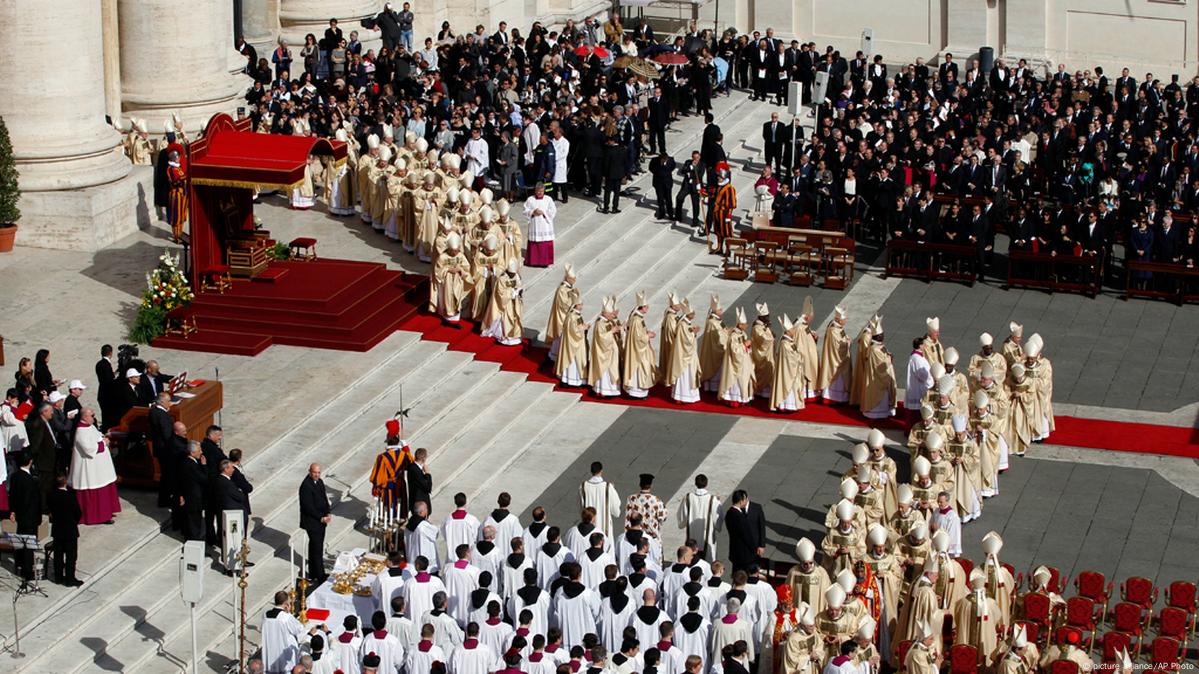This detailed aerial image captures an elaborate outdoor Catholic ceremony taking place in front of a grand, large building that appears to be a church. The facade of the building is adorned with very large white pillars and a grand set of stone steps that lead up to a stage altar. The altar is extravagantly decorated with red elements, including steps, seats, background, awning, and a carpet that extends down the steps onto a designated pathway.

The focus of the image is a solemn procession of religious officials, clad in their distinctive attire of white and gold robes, as well as shiny beige robes. These officials, possibly priests, cardinals, or deacons, are seen walking in a structured line down the red carpeted steps. The procession weaves from the bottom left of the image, extends towards the right, then crosses horizontally through the center up to the upper left, creating a striking visual.

This procession is observed by a large gathering of spectators, all dressed in formal black attire, primarily black suits, seated and standing around the pathway. The spectators also populate the background, especially on the middle upper left side and along the upper portion of the image, creating an atmosphere of deep reverence and anticipation. The entire scene is illuminated by bright daylight, adding a layer of solemnity and clarity to this significant religious event.